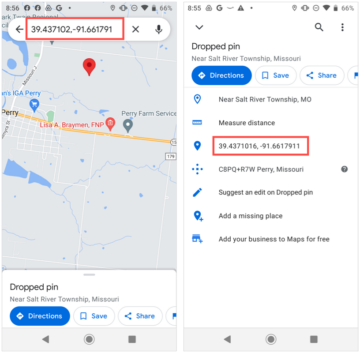The image showcases a detailed map section, prominently featuring a location marked by a pin. On the left side, a map identifies the location labeled "Lisa A. Brayman, FNP Perry Farm Service." Below this map, text reads "Dropped pin near Salt River Township, Missouri." Further below, it offers options for "Directions," "Save," and "Share."

On the right side, an elongated rectangle reiterates the dropped pin's information, stating "Dropped pin near Salt River Township, Missouri." However, the text "near Salt River Township, Missouri" appears blurry and smaller in font size compared to "Dropped pin." Beneath this is another set of options: "Directions," "Save," and "Share." The section concludes with vertically aligned text reading "near Salt River Township, MO" and "Measure distance."